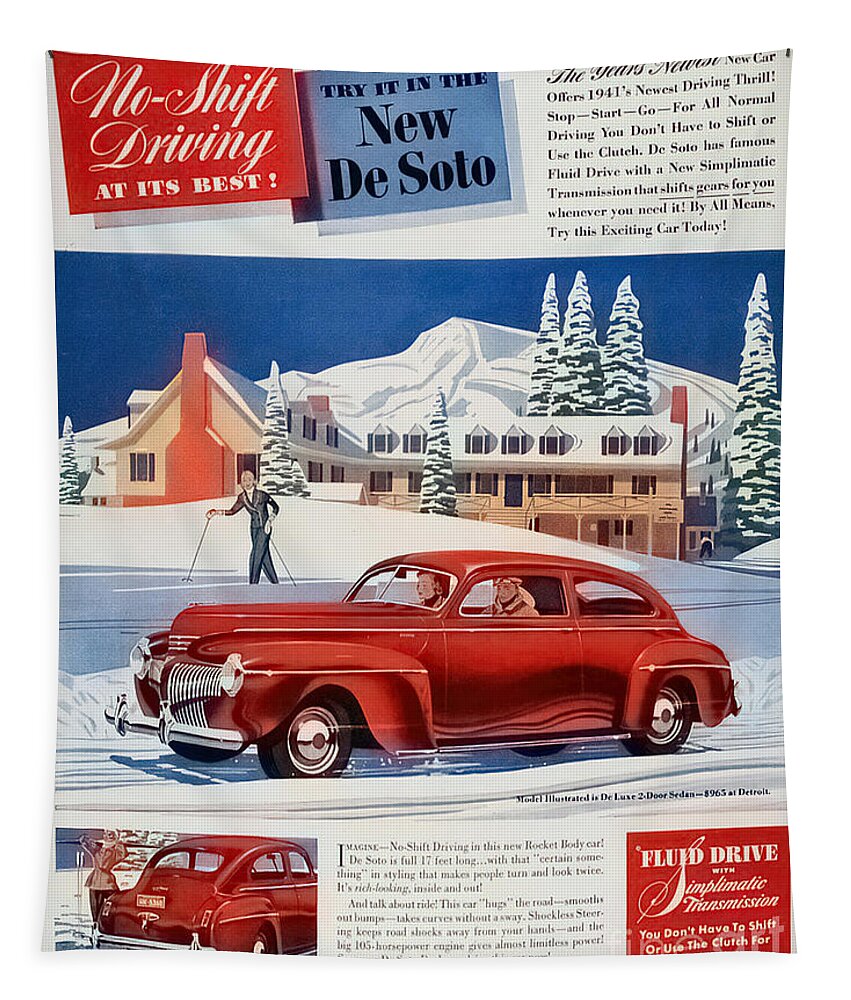This vibrant and nostalgic advertisement, likely from the 1940s or early 1950s, showcases the new DeSoto automobile with its groundbreaking no-shift driving experience. The headline at the top, written in elegant white script on a red background, proudly proclaims "No Shift Driving at its Best." Below, in a bold blue box with black lettering, it invites you to "Try it in the new DeSoto."

The advertisement features a detailed illustration centered around a winter ski resort. Snow-covered mountains and conifer trees set a picturesque backdrop, with a charming yellow-and-orange ski lodge nestled in the scenery. A man, clad in a black ski suit, poses with skis in hand, ready to hit the slopes.

Dominating the foreground is a striking red DeSoto sedan, its long front and bubble-like roof capturing the essence of mid-century automotive design. Inside the car, a lady with blonde hair sits behind the wheel, accompanied by a man. Chrome details gleam, highlighting the car's stylish and modern features.

To the right of the scene, additional advertising copy emphasizes the vehicle’s advanced features, such as "Fluid Drive" and "Symptomatic Transmission." At the bottom edge, another image of the car showcases its rear view, reinforcing the sleek design and elegance of the DeSoto. This colorful, vintage ad not only promotes a car but also captures the innovative spirit of its era.